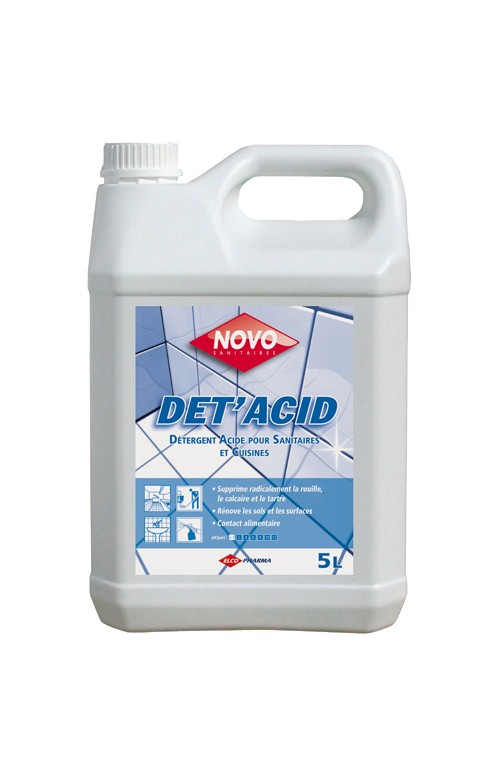The photograph features a large, opaque white plastic jug with a horizontal handle on the top right and a circular ribbed white cap on the top left. The jug is designed for sanitary cleaning, specifically a detergent labeled as "DET Acid” (with an apostrophe between DET and Acid), noting its acidic properties for bathroom and kitchen use. Positioned prominently in the center of the jug is a vertical rectangular label. The top of this label displays a horizontal red diamond containing the word "NOVO" in large white letters. The label’s background includes a depiction of a clean, shining bathroom floor and tiles.

Below the NOVO logo, the product name "DET Acid" is written in capital blue letters with a white outline. Directly underneath, the text "DETERGENT ACID POUR SANITARE A GUISINE" (French for acidic detergent for sanitary and kitchen use) appears. Further down, there is a blue horizontal bar with four small squares illustrating various images including a washbasin, a man mopping, a clean floor, and possibly a shower area. To the right of these images, a series of bullet points in white text provide product usage instructions in French, detailing its powerful cleaning abilities ("supreme radical amendment," "la rouille les calcaires et les tartres," "renover les sols et les surfaces," and "contact élémentaire"). 

Additionally, at the bottom center of the label, there's another red diamond logo featuring the brand "ELKO" in white letters, with "PHARMA" written beneath it. In the bottom right corner of the label, the quantity "5L" (5 liters) is clearly marked, indicating the volume of the contents. The background of the image consists of clean white tiles interspersed with blue tiles, adding to the sanitary setting of the product.